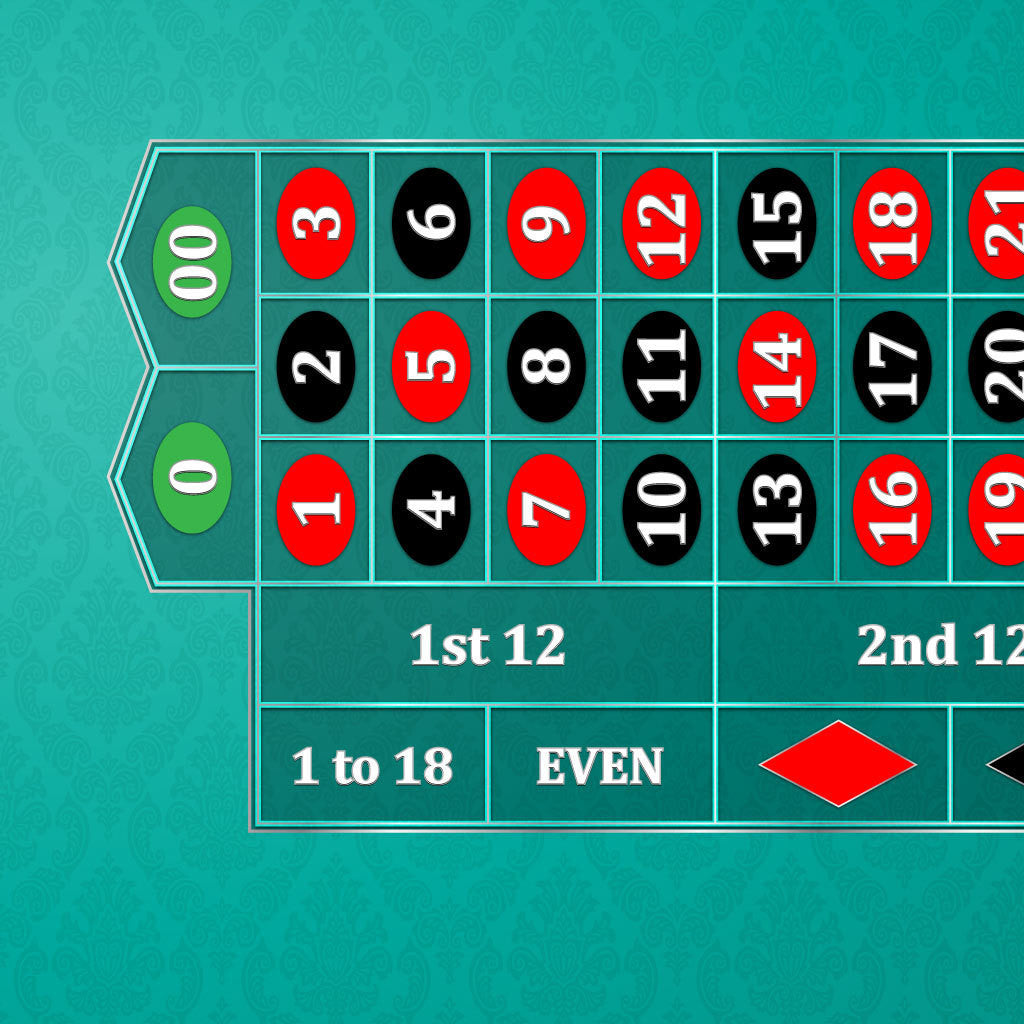The image portrays a close-up, overhead view of a roulette betting board with a bluish-green felt background, adorned with an intricate, darker bluish-green pattern overlay. The focus is on the left part of the table, which prominently features a home base pentagon shape on the left side, containing two green ovals marked with a zero and double zeros. A horizontally-aligned, grid-like pattern extends from this pentagon, filled with red and black ovals signifying different numbers. The red ovals include 1, 3, 5, 7, 9, 12, 14, 16, 18, 19, and 21, while the black ovals feature numbers such as 2, 4, 6, 8, 10, 11, 13, 15, 17, and 20. 

Below this grid, rectangular sections indicate betting ranges: the first section states "First 12," "1 to 18," and "Even," while the second section states "Second 12," and includes red and black diamonds, representing additional betting options. The board’s right edge is cut off, restricting the visible area to the detailed left side of the roulette layout.